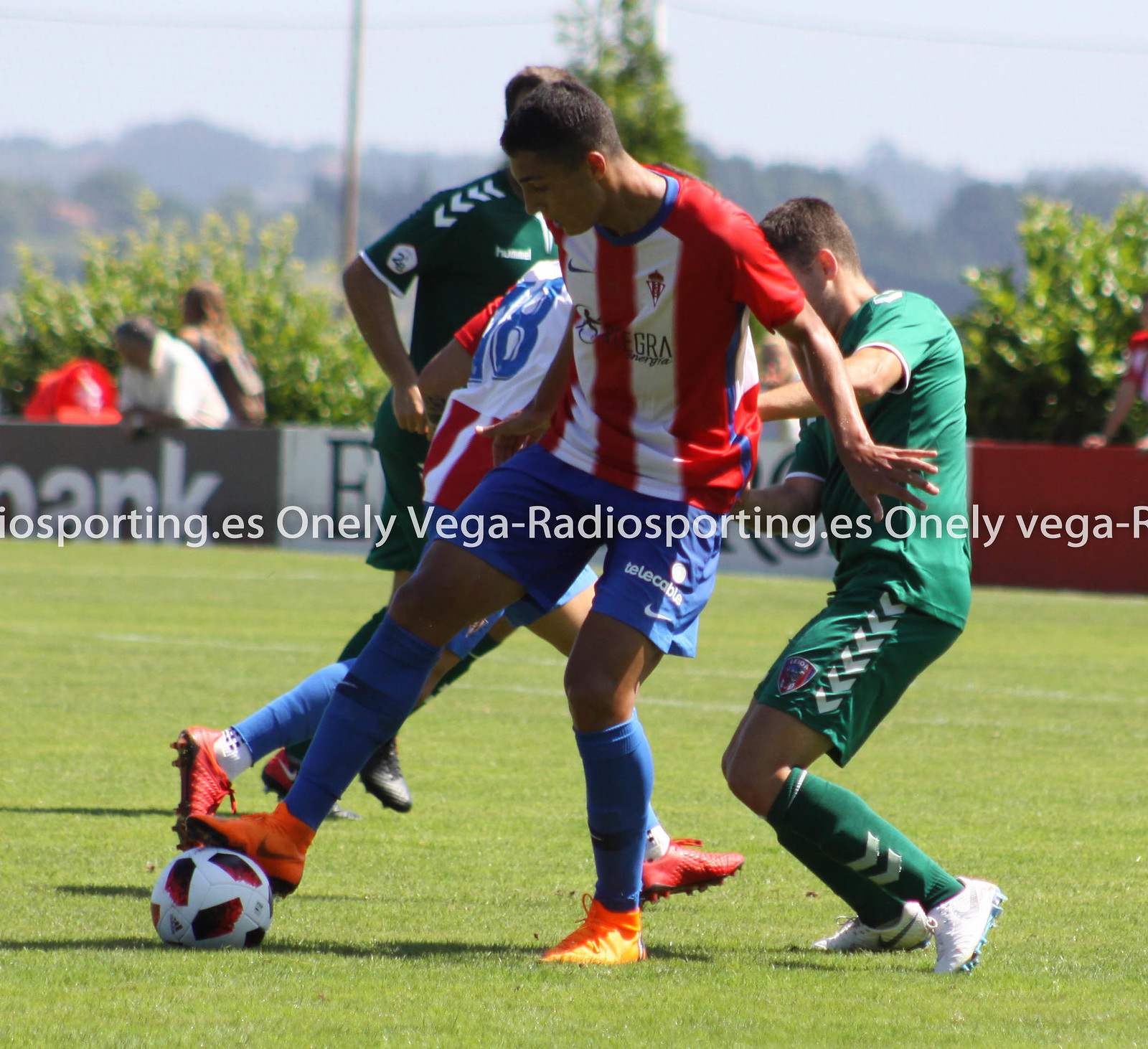This full-color, square photograph captures the dynamic action of a soccer match in broad daylight with four central players. Two of the players are wearing red and white vertically striped shirts with blue shorts and blue socks, sporting orange shoes, while the other two players are clad in all-green outfits with matching green shirts, shorts, and socks, along with white shoes. They are fiercely competing for a white soccer ball that features red and black accents. The lower half of the background prominently showcases green grass, while the upper half reveals an out-of-focus scene with trees and what appears to be mountains under a clear blue sky. Additionally, there are a few indistinct spectators near the edge of the field. The image also features several texts and signs, including "GoSporting.es", "OneLeague", and "Vega Radiosporting.es", which suggest related websites and media. A superimposed watermark is present over the entire center of the photograph.